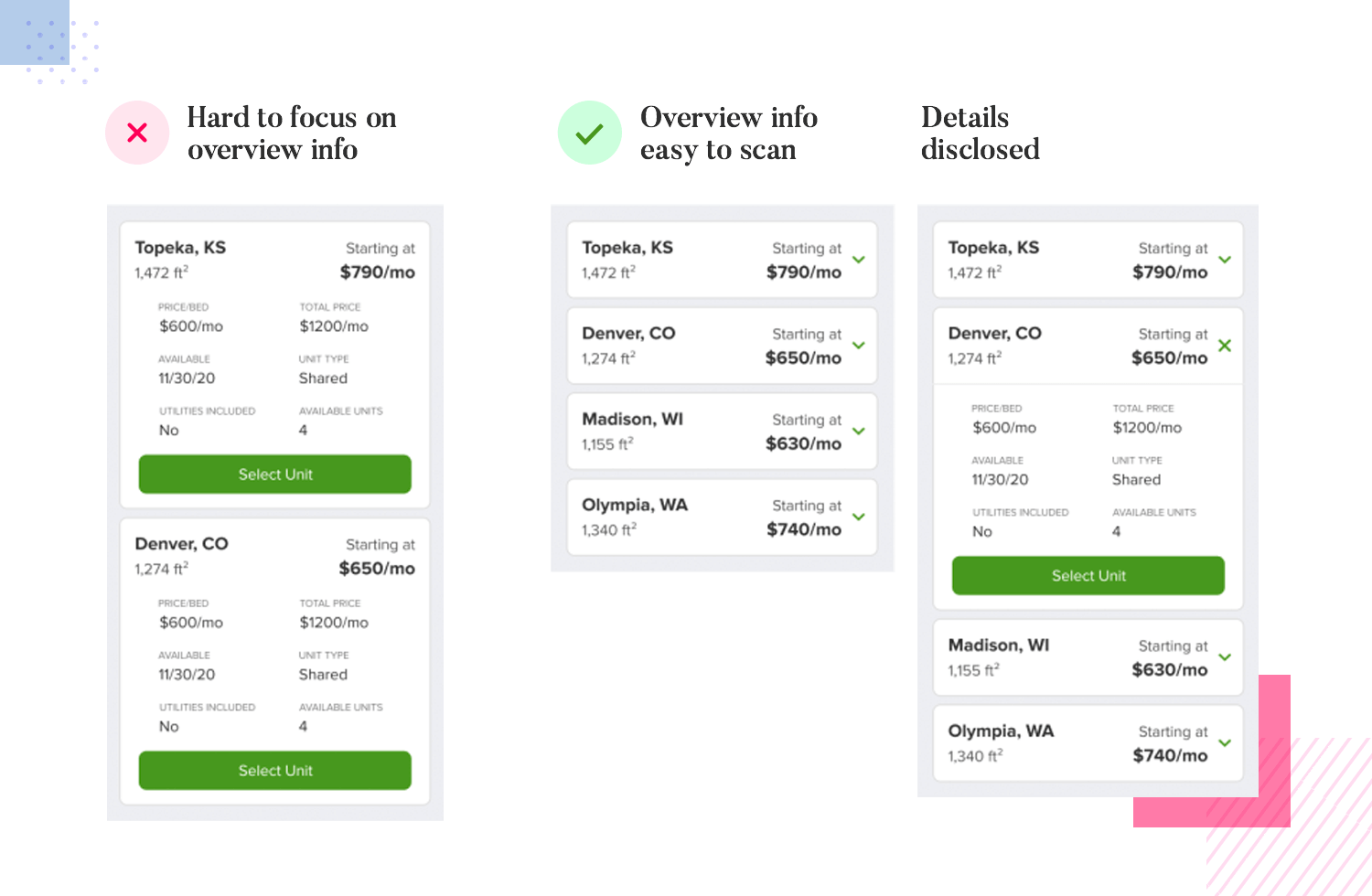A screenshot with a white background features a blue square in the upper left-hand corner. Within this blue square is another one, positioned slightly to the right and above, which is made up of smaller blue dots, clearly forming a square shape.

Beneath this, there are three headers:
1. On the left, a light pink circle with a red X inside is next to the bold text "Hard to Focus on Overview Info."
2. In the center, a pastel green circle with a green check mark inside is next to the bold text "Overview Info Easy to Scan."
3. On the right, the bold text "Details Disclosed" serves as the label for the third column.

Under each header, gray-outlined rectangles with white centers are arranged. Under "Hard to Focus," there are two entries:
- Topeka, Kansas
- Denver, Colorado

Under "Overview Info Easy to Scan,” there are four entries:
- Topeka, Kansas
- Denver, Colorado
- Madison, Wisconsin
- Olympia, Washington

Under "Details Disclosed," there are also four entries, with one expanded to be slightly larger:
- Topeka, Kansas
- Denver, Colorado (expanded)
- Seattle, Washington
- Madison, Wisconsin
- Olympia, Washington

In the lower right-hand corner of the image, a thick, hot pink backwards 'L' marks the corner, adding a distinct visual marker.